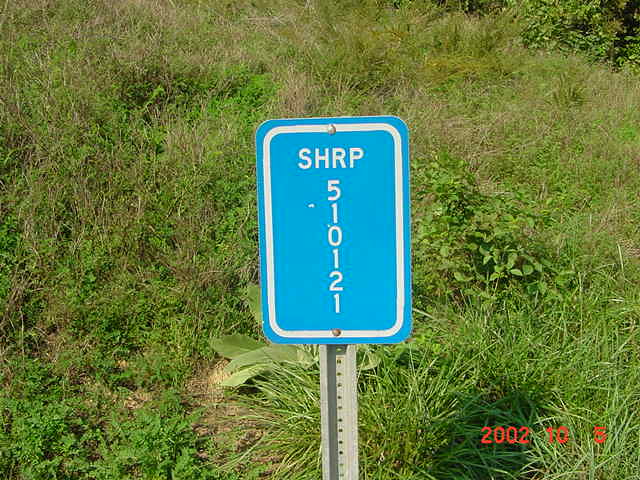A sky blue, vertically rectangular sign with a white trim stands prominently at the edge of a road, amid lush green foliage interspersed with some withered bushes. The sign, which does not appear to demarcate a highway or function primarily for pedestrian use, displays the acronym "SHRP" at the top. Below this, the sequence "510121" is written vertically from top to bottom. At the bottom of the sign, the number "200210" is clearly visible, along with an additional, partially legible number. The scene suggests a slightly elevated location, contributing to its notable, though not urgent, relevance.